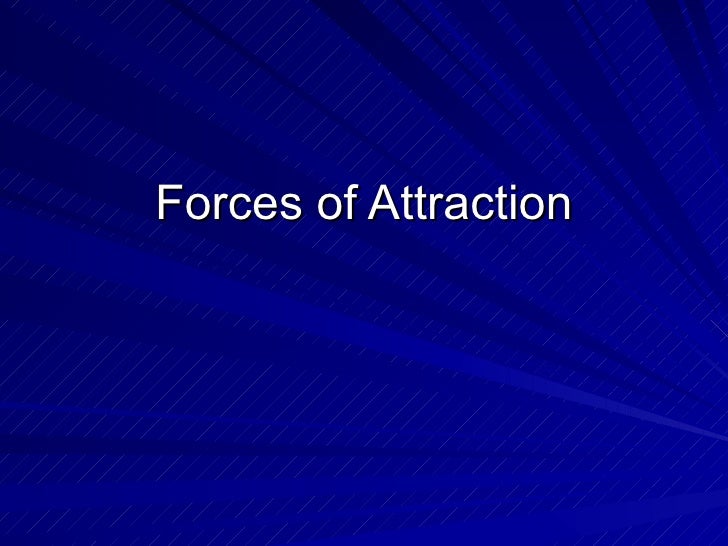The image is a still from a PowerPoint presentation slide featuring a simplistic design with a blue gradient background. The gradient transitions from a darker blue in the top left to a lighter blue in the bottom right, creating a sunburst or fan-like pattern emanating from the bottom right corner. The background includes a mix of blue hues with darker blue waves and perpendicular, thin white lines adding texture. Prominently centered on the slide in slightly raised Arial font, the white text reads "Forces of Attraction" with a slight black drop shadow for emphasis. The words "Forces" and "Attraction" are both capitalized.